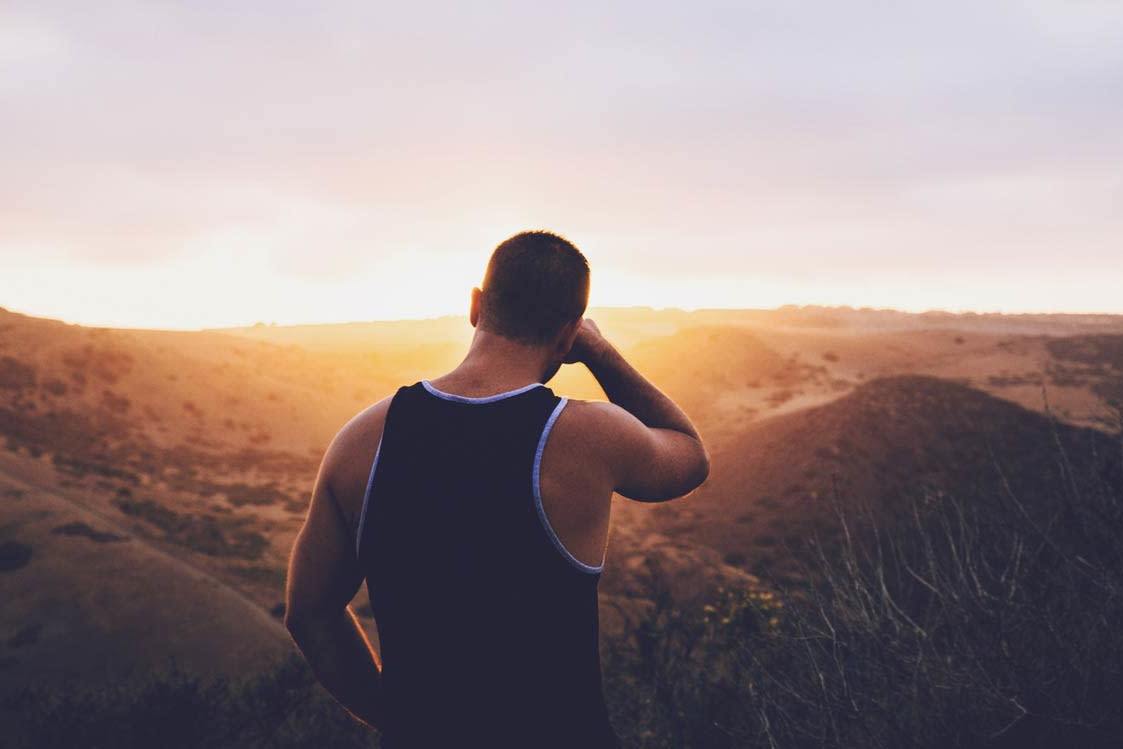The image captures a muscular man with short, almost buzzed hair, standing in a vast, dry sandy landscape, possibly a desert with hilly terrain. The sun is setting, casting a wide, golden glow across the scene. The man, viewed from behind, is wearing a black sleeveless tank top with distinctive white trim around the neckline and armholes. He is blocking the direct rays of the sun with his right hand, raised in front of his face, perhaps to shield his eyes. His left arm hangs naturally at his side. He stands solemnly, facing the horizon, seemingly lost in the beauty of the sunset or deep in introspection. There are no buildings or other structures, emphasizing the isolation and expanse of the landscape.